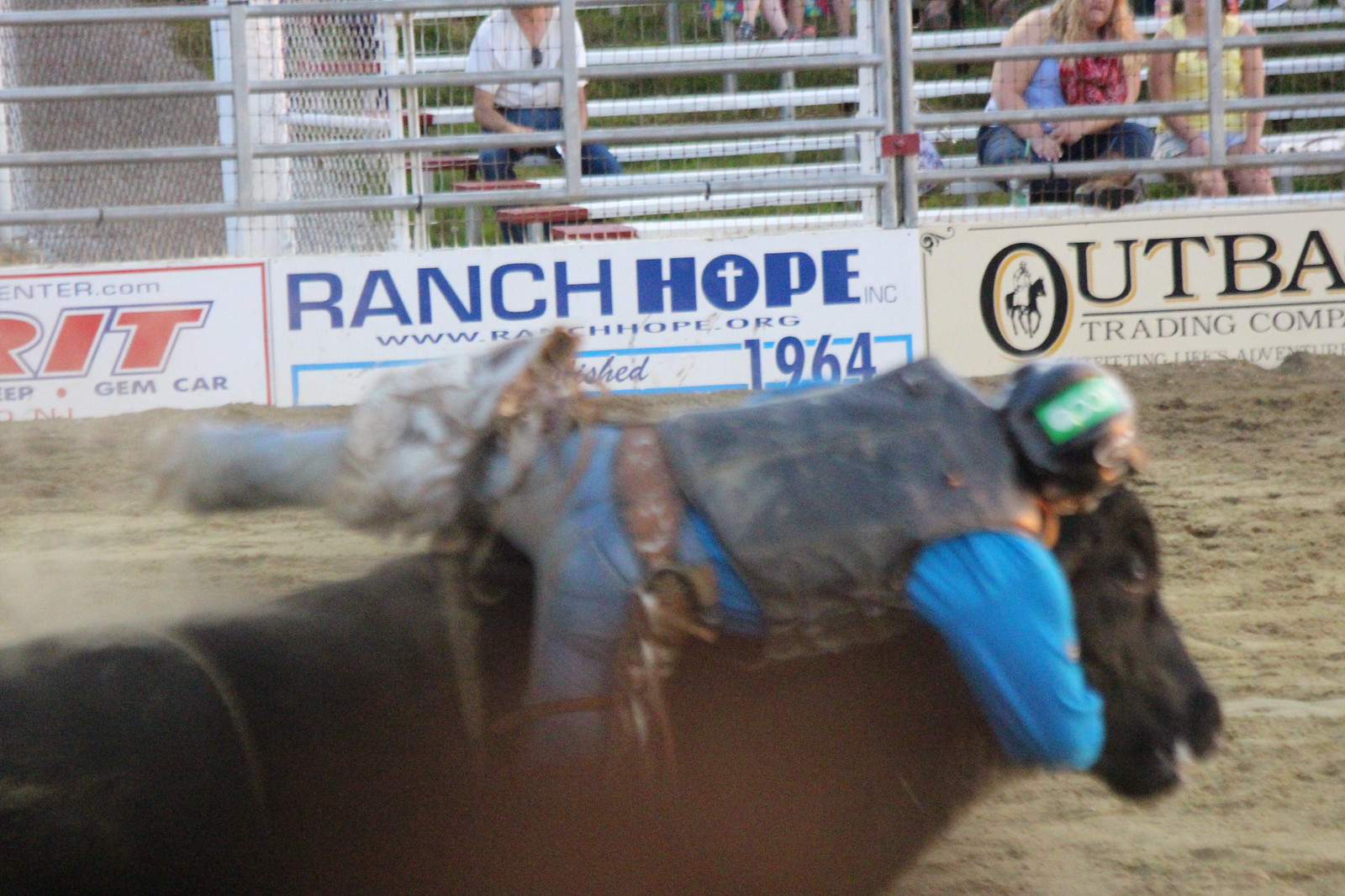A dynamic action shot captured at a rodeo, featuring a black bull at the bottom left and middle of the image with a rider clinging to its neck. The rider, who is bracing himself to avoid being thrown, is equipped with a protective black leather vest, a long-sleeved blue shirt, light denim blue jeans, and chaps, with leather pieces dangling off him. His torso is protected by a shield, and he's wearing a helmet. The bull and rider are seen charging through a dirt, sandy arena, their blurred motion conveying the intensity of the moment. Surrounding the arena, the fence line is dotted with advertisements, including ones for Ranch Hope (www.ranchhope.org, established 1964) and Outback Trading Company. Beyond the fence, spectators can be seen watching the action unfold, with their eager faces adding to the energy of the scene.